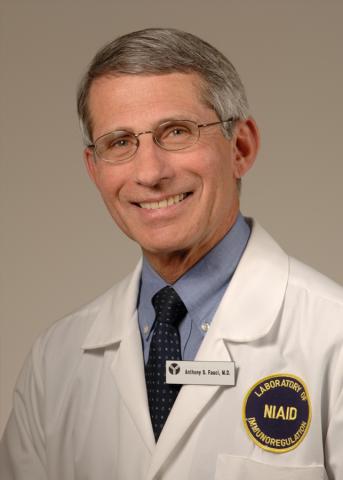This is an old photograph of a somewhat younger Dr. Anthony Fauci, likely in his 50s, sitting in front of a beige background and smiling. He is wearing a white lab coat adorned with a black and yellow patch that reads "Laboratory of Immunoregulation, NIAID." The name tag on his collar says "Anthony B. Fauci, MD." Underneath the lab coat, he has on a collared blue shirt and a blue tie with white polka dots. Dr. Fauci's hair is beginning to turn gray at the sides and is neatly combed over. He is also wearing round glasses.